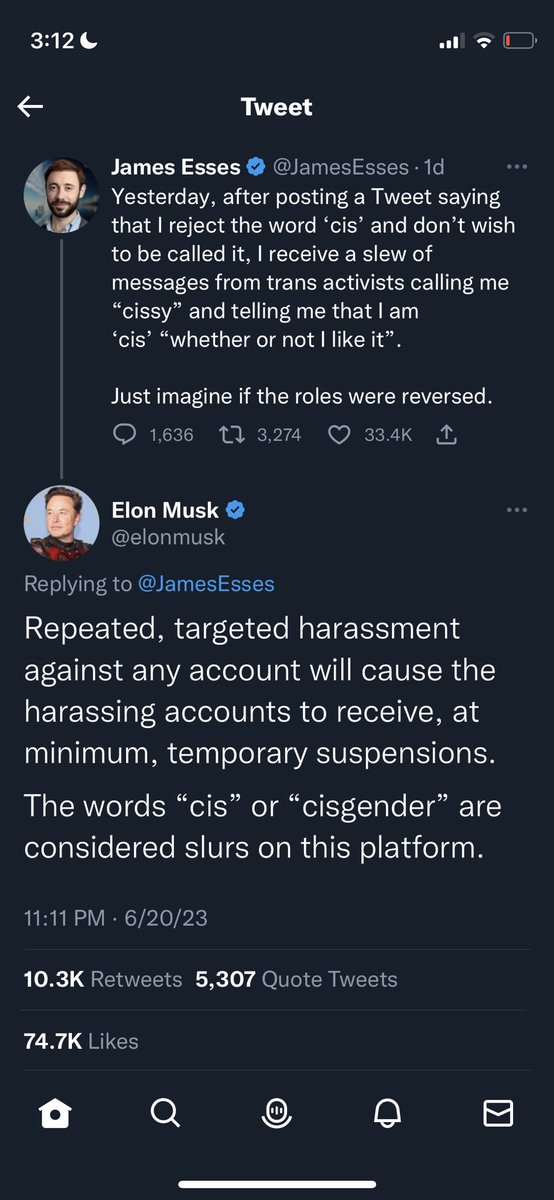This image is a mobile screenshot of a Twitter exchange featuring a notable interaction. The background is a dark bluish-gray color, indicating that the screenshot was likely taken in night mode, and the device's battery icon shows low charge in red. Captured at 3:12 with a moon icon present, implying it was taken either late at night or early in the morning.

At the center of the exchange is a tweet from James Esses, a white man with brown hair and a beard. His tweet, posted one day ago, reads: "Yesterday, after posting a tweet saying that I reject the word ‘cis’ and don't wish to be called it, I received a slew of messages from trans activists calling me 'sissy' and telling me that I am ‘cis’ whether or not I like it. Just imagine if the roles were reversed." This tweet has garnered significant attention, amassing 1,636 comments, 3,274 retweets, and 33,400 likes.

In response to James Esses’ tweet, Elon Musk replied: "Targeted harassment against any account will cause the harassing accounts to receive at minimum temporary suspensions. The words ‘cis’ or ‘cisgender’ are considered slurs on this platform." Musk's reply, posted at 11:11 PM on June 6, 2023, has also attracted substantial interaction, with 10.3K retweets, 5,307 quote tweets, and 74,700 likes.